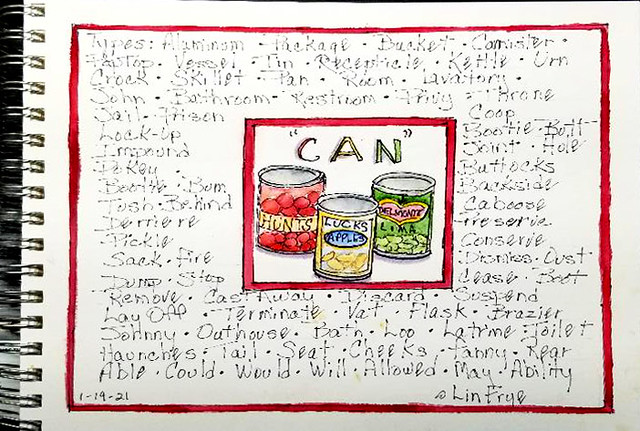The image displays a detailed colored photograph of a drawing on a white sheet of paper secured in a silver spiral binder, with the spiral visible on the left side. The drawing is bordered by a thin red rectangle. Inside, the word "can" appears prominently in green with quotation marks around it, situated within another rectangle in the center. Below this are three illustrated cans, each distinctly colored and labeled. The can on the left is marked with a red and yellow logo, reading "Banner Hunts." The middle can features a yellow and blue design with "Lux Apples" inscribed on it. The can to the right has a green label and reads "Del Monte Lima." Additional pencil annotations, though faint and broken, are scattered around the image, describing various can types and packaging. In the lower corners of the paper, there is a date "1-19-21" and what appears to be a signature, "LINFRYE," in the lower right.